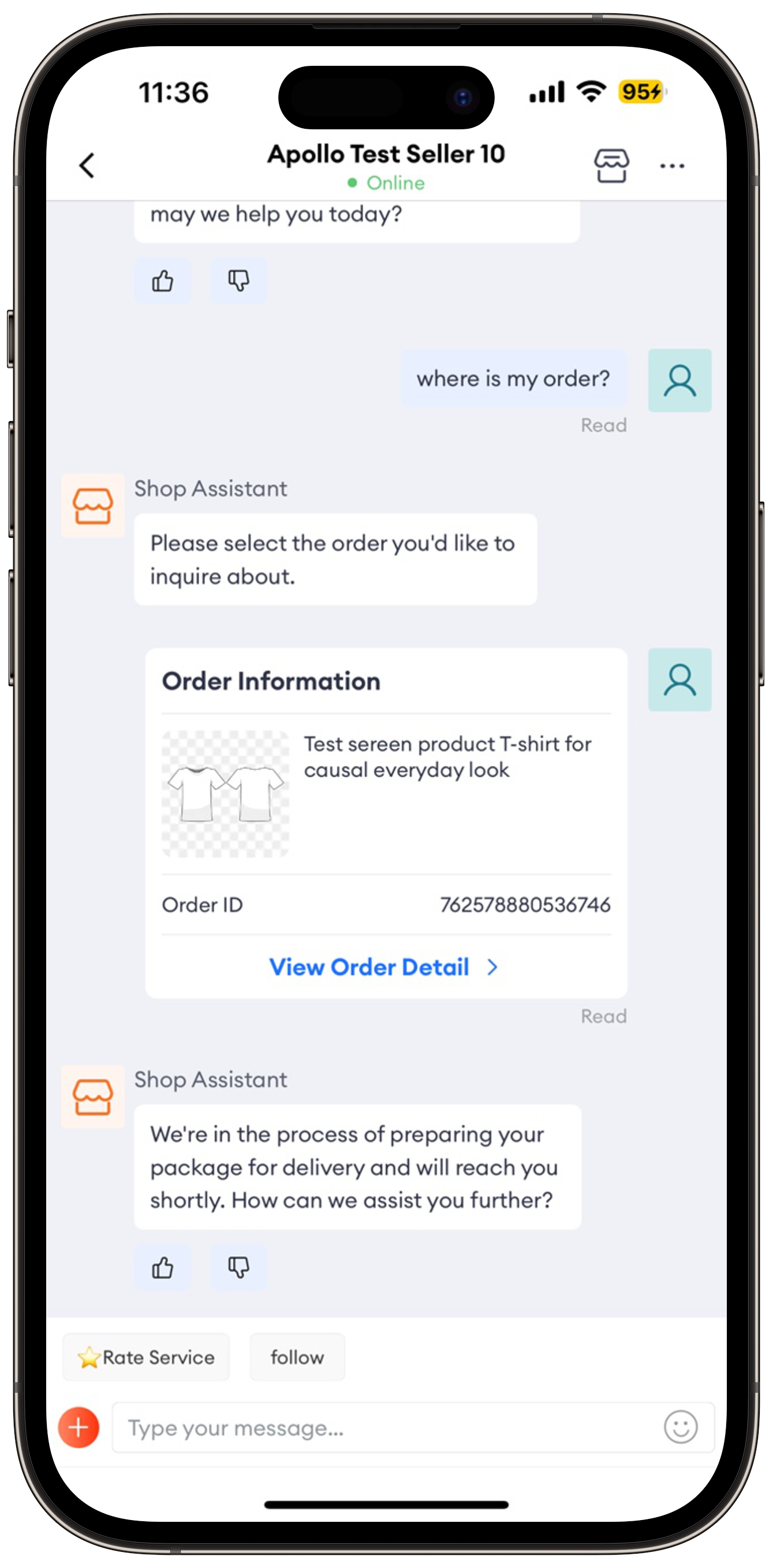This image showcases a mobile device, prominently displaying an ongoing conversation on its screen. The device, encased in a sleek black plastic cover, is set against a clean white background, accentuating its front display.

### Details of the Display:
- **Status Bar** (Top of the screen):
  - **Time:** 11:36, displayed in black on a white background.
  - **Signal Strength:** Full bars (4 out of 4).
  - **Wi-Fi Connection:** Full signal.
  - **Battery Indicator:** 95% battery life with a lightning bolt symbol inside a yellow rectangle.

- **Front Camera**: A small circular lens positioned centrally just below the status bar.

- **Header Information**:
  - **Text:** "Apollo test seller 10 online".
  - **Icons**: 
    - **Left**: A back or "less than" symbol (<).
    - **Right**: Archive symbol and a three-dot menu icon.

- **Main Content**:
  - A light grey background hosts a conversation interface.
  - **Message Threads**:
    - **First Message (Left Aligned)**: A partial message ending with "may we help you today?" followed by thumbs up and thumbs down icons.
    - **Second Message (Right Aligned)**:
      - **Text:** "where's my order?" in lowercase.
      - **Symbol**: A blue icon of a person within a lighter blue square, indicating the message’s reading status ("read").
    - **Third Message (Left Aligned)**:
      - **From:** Shop assistant, represented by a light orange circle with an orange shop icon.
      - **Text:** "please select the order you'd like to inquire about."
    - **Fourth Message (Right Aligned)**:
      - **Text:**
        - "Order information:"
          - Product description: "test screen product t-shirt for casual everyday look".
          - Icons of t-shirts on a transparent grid.
          - Order ID: "762578880536746".
          - Action: "View order detail", marked as read.
    - **Fifth Message** (Left Aligned):
      - **From:** Shop assistant.
      - **Text:** "we’re in the process of preparing your package delivery and we'll reach you shortly. How can we assist you further?" followed by thumbs up and thumbs down icons.
      - **Buttons:** "Service" and "Follow".
  - **Bottom Section**:
    - **Input Field:** "Type your message" placeholder for user input.
    - **Icons**:
      - **Left:** Red circle with a plus sign.
      - **Right:** Emoji icon.

This highly detailed view captures the functional interface of a messaging conversation on the mobile device, portraying various elements of interaction between the user and a shop assistant within a shopping or service application.